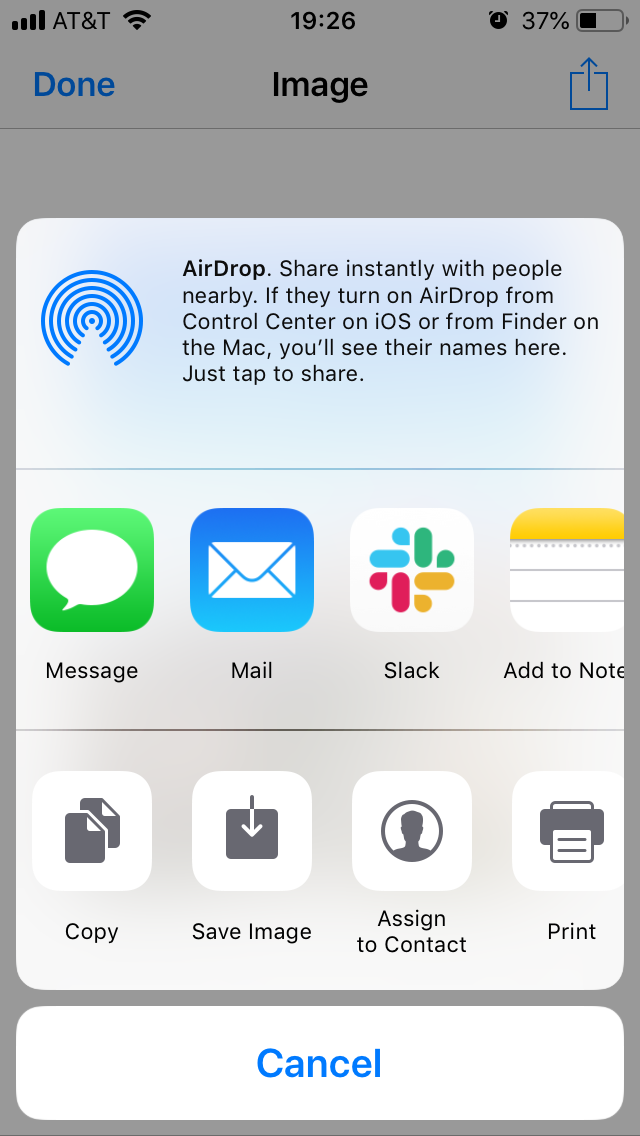Here is a cleaned-up and detailed caption for the described image:

---

A detailed screenshot of an iPhone, showing a partially grayed-out background with a white pop-up window in the foreground. The background reveals key device details: a full four bars of AT&T network coverage, Wi-Fi connection active, the time displayed as 19:26, and the battery level at 37%. 

At the top of the white pop-up window, the title "AirDrop" is visible, accompanied by an explanatory text: "Share instantly with people nearby. If they turn on AirDrop from Control Center on iOS or from Finder on the Mac, you'll see their names here. Just tap to share." This text is complemented by an icon on the left depicting concentric circles with a bottom wedge missing.

Directly underneath, a row of sharing options is available, featuring icons labeled MESSAGE, MAIL, SLACK, ADD TO NOTES, COPY, SAVE IMAGE, ASSIGN TO CONTACT, and PRINT. The lower section of the pop-up includes a white rectangular button with "CANCEL" written in blue letters.

This screenshot contains no photographic elements, people, animals, or natural elements like plants, flowers, or trees, focusing entirely on the interface and functionality of the AirDrop feature on the iPhone.